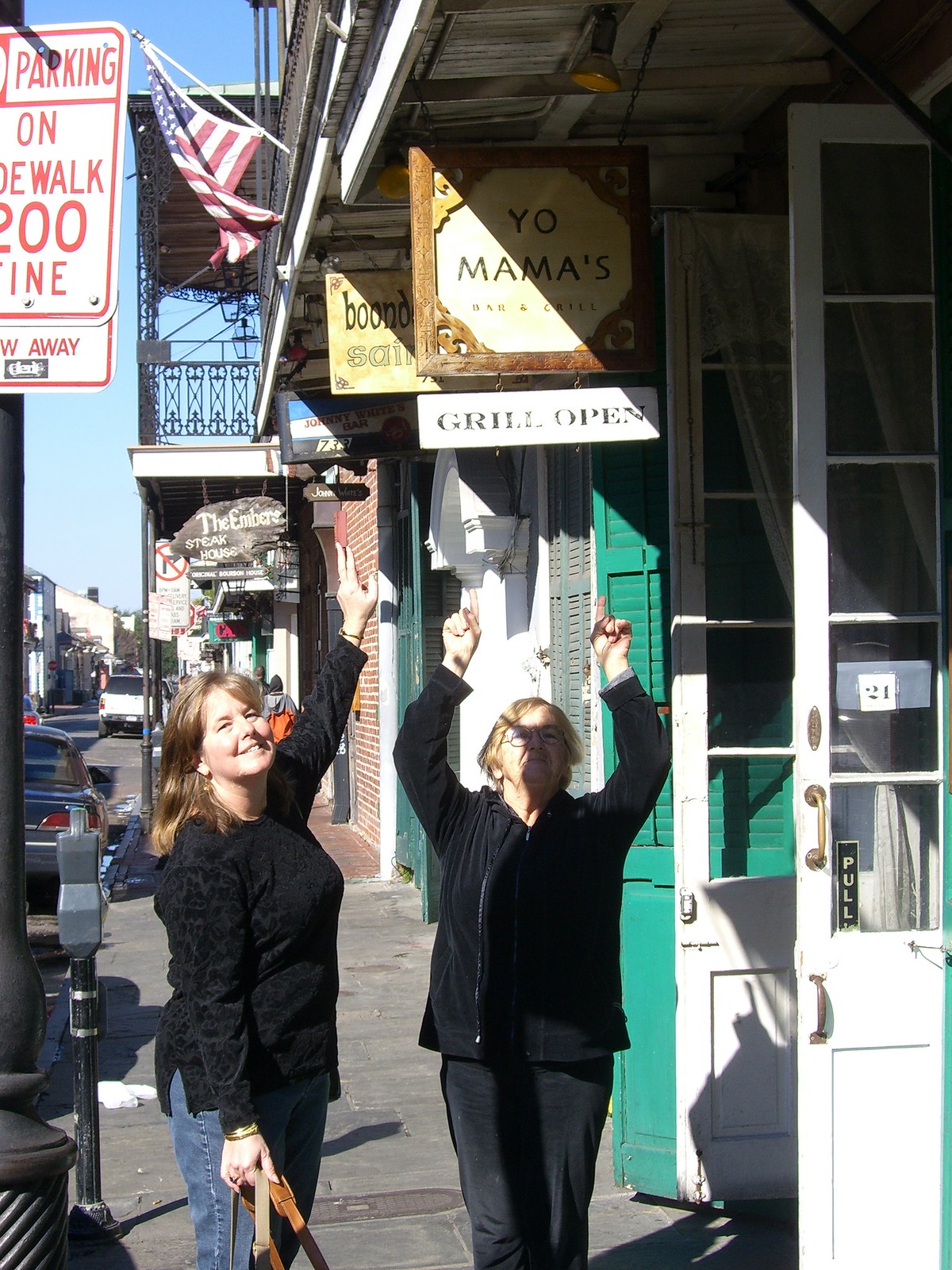In a bustling cityscape reminiscent of a charming market area in the United States, a photo captures a vibrant moment on a sidewalk lined with various small shops and awnings. The scene is framed by a parking sign in the top left corner, next to an American flag gently waving in the breeze. Below, the street is edged with parked cars and punctuated by a parking meter. 

The focal point of the image is two women standing on the sidewalk, directly beneath a sign that reads "Yo Mama's Bar and Grill - Grill Open." The woman on the left, dressed in a black shirt and holding a bag, is likely around her 30s, with long brown hair. Next to her is an older woman, possibly in her 50s or 60s, wearing glasses, a black sleeveless jacket, and black pants. Her blondish hair matches the color of the younger woman's, hinting at a familial relationship, likely mother and daughter. Both are enthusiastically pointing up at the "Yo Mama's" sign, engaging in a playful moment.

The background reveals brick walls and open wooden doors painted white, enhancing the quaint, inviting ambiance of the scene. Together, these elements create a lively snapshot of city life, highlighting the bond between the two women and their shared sense of humor.